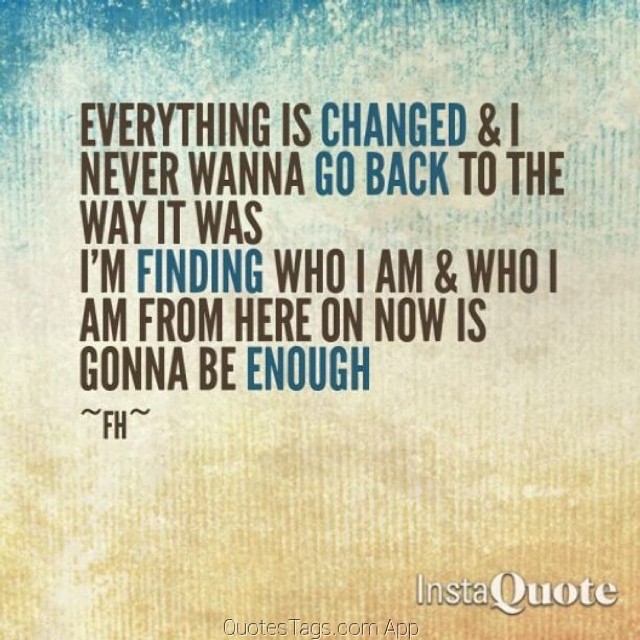This image appears to be a digitally designed card, divided into two sections with a blue and white gradient on the upper half and a light brown and white gradient on the lower half. At the center of the image, there's a motivational quote, presented in six lines of capitalized text: "EVERYTHING IS CHANGED AND I / NEVER WANT TO GO BACK TO THE / WAY IT WAS / I'M FINDING WHO I AM AND WHO I / AM FROM HERE ON NOW IS / GOING TO BE ENOUGH." Most of the text is in a dark brown color, with the words "CHANGED," "GO BACK," "FINDING," and "ENOUGH" highlighted in blue.

Beneath the text, on the left side, there are two squiggly lines with the initials "FH" between them. In the bottom right corner, the text "InstaQuote" is written in larger white letters. Additionally, at the bottom center, the watermark "cutetext.com app" appears in faint writing. The overall design and text placement suggest that this image is intended for use as an inspirational post, suitable for sharing on social media.